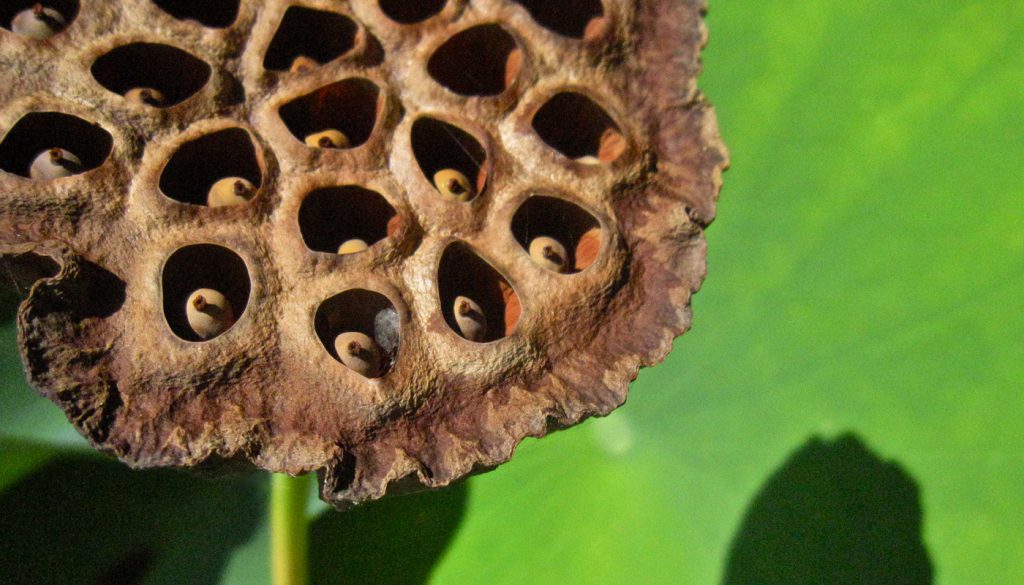The image depicts a mature seed pod positioned in the upper left corner, showcasing a circular structure with jagged, crimped edges resembling a pastry. The outer edges of the pod are dark brown, transitioning to a lighter brown and yellow tint towards the center. Each circular opening within the pod contains a round tan seed with a darker brown spot prominently atop it. Some seeds appear shadowed and dark, while others on the right side catch a bit of light, revealing a lighter amber hue at the bottom. In the central spaces between these circular pods, hints of white and light yellow can be seen. The uppermost openings reveal no visible seeds, only light shining through, particularly noticeable in three openings at the top right. The pod is mounted on a green stem, set against a backdrop of what seems to be a large green leaf that casts various shadows. Darker shadows are prominent beneath the flower, especially on the bottom left side and beneath the pod itself.